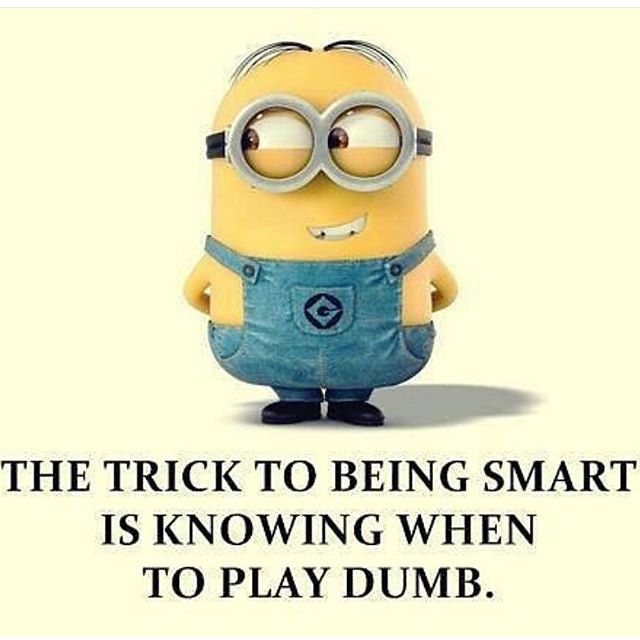The image is an inspirational meme with a light yellow background featuring a cartoon 3D-rendered creature resembling a Minion from Despicable Me. The creature is bean-shaped and entirely yellow, wearing blue jean overalls adorned with a circular logo with a 'G' in the center. It has two large, white eyes with brown irises that are covered by round, silver-rimmed goggles with a black band. The Minion's gaze is directed to the left, and it has a few strands of black hair emerging from the center of its semi-bald head. With its hands behind its back and a slight smile on its face, the Minion completes its look with black shoes. Below this character, written in black all-capital letters, is the quote: "THE TRICK TO BEING SMART IS KNOWING WHEN TO PLAY DUMB."